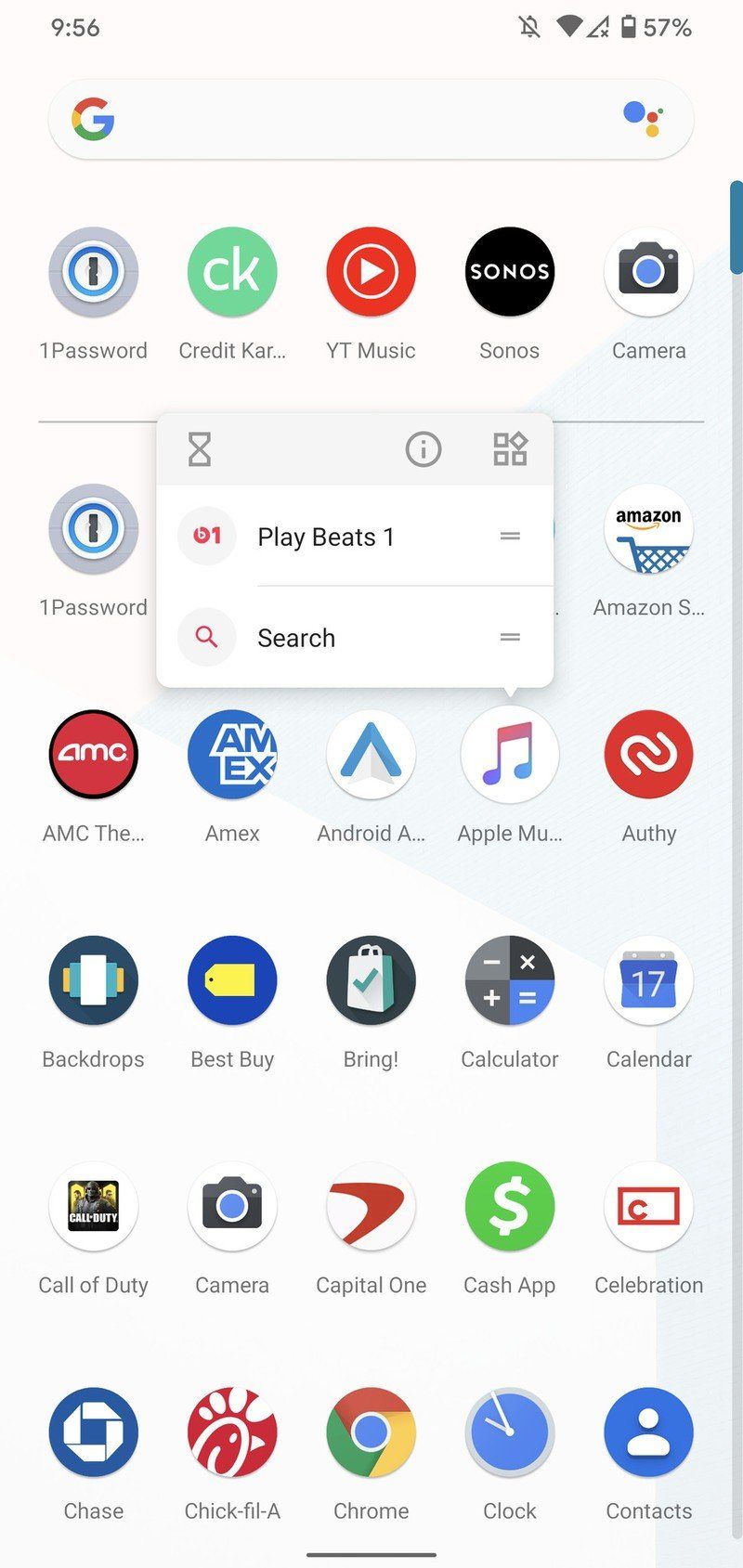The image depicts the home screen of a likely Android device, possibly a Google Pixel, given the presence of a Google search bar. The background is characterized by a subtle white gradient transitioning into light blue hues. The status bar at the top shows the time, 9:56, with the sound muted, full Wi-Fi signal, no network signal, and a battery level at 57%.

Prominently displayed in the foreground is a pop-up box from Apple Music, offering options such as "Play Beats 1" and "Search," indicating that this app has been interacted with recently.

In the background, the device's home screen is densely populated with a multitude of apps, including but not limited to:

- 1Password
- Credit (suggesting a finance-related app)
- K-I-A-R
- YouTube Music
- Sonos
- Camera
- Amazon Store
- AMC (likely related to entertainment or cinema)
- American Express (Amex)
- Android-related apps (Android A)
- Authy (security/authentication app)
- Best Buy
- Bring (possibly a shopping list app)
- Calculator
- Calendar
- Call of Duty (a game)
- Capital One
- Cash App
- Celebration (unknown, possibly an event-related app)
- Chase Bank
- Chick-fil-A
- Chrome browser
- Clock
- Contacts

The organized layout and the variety of app categories suggest a user who utilizes their device for a wide range of activities, from entertainment and shopping to finance and utilities.